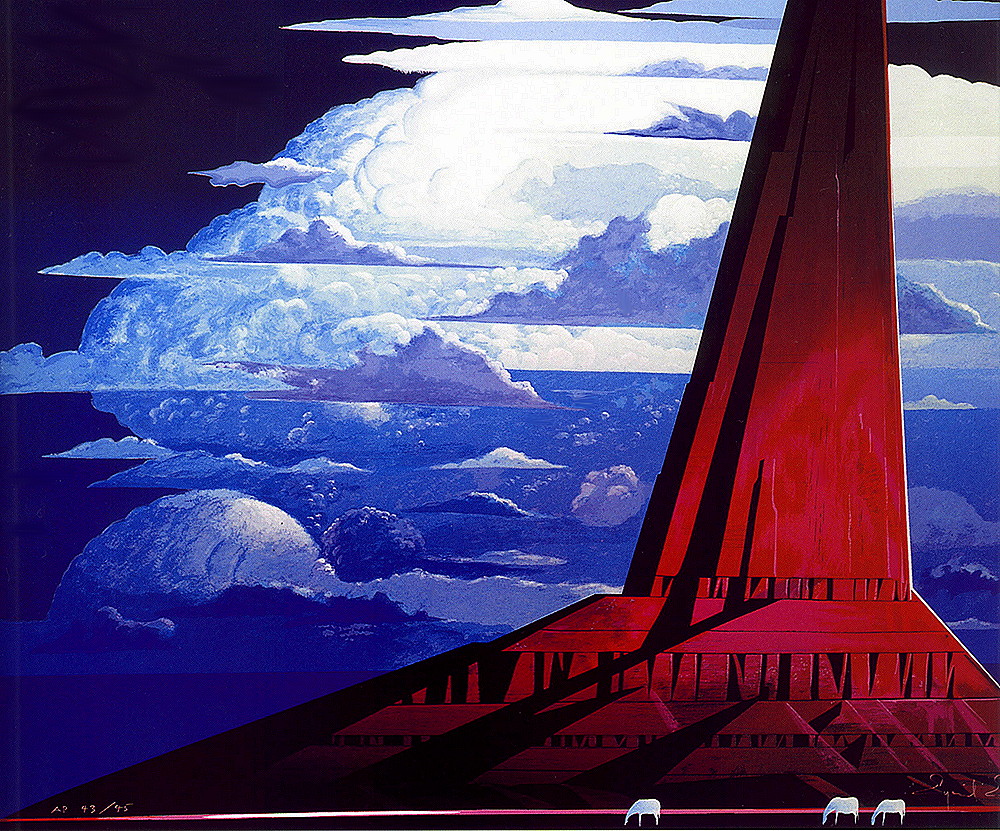This detailed painting, possibly digital artwork, captures an evocative outdoor scene. The focal point is a striking, reddish structure with an industrial aesthetic, possibly resembling a vessel or architectural feature. It has a triangular base that extends upward and off the frame, adorned with black shadows and intricate lines. Set against this is a dark night sky interspersed with puffy cumulus clouds, ranging from brilliant white to shades of blue, possibly reflecting the sea below.

In the foreground, three small, blue sheep, stylized and with minimal detail, graze on the dark ground, trailing from the right to the left in profile. The contrasting colors of red, black, and blue dominate the composition, drawing viewers into the depth of the scene. The painting also includes an artist's signature in the lower left-hand corner, though it's unreadable.

Overall, this painting melds elements of nature and man-made structures in a captivating, surreal tableau rich in texture and color variations.